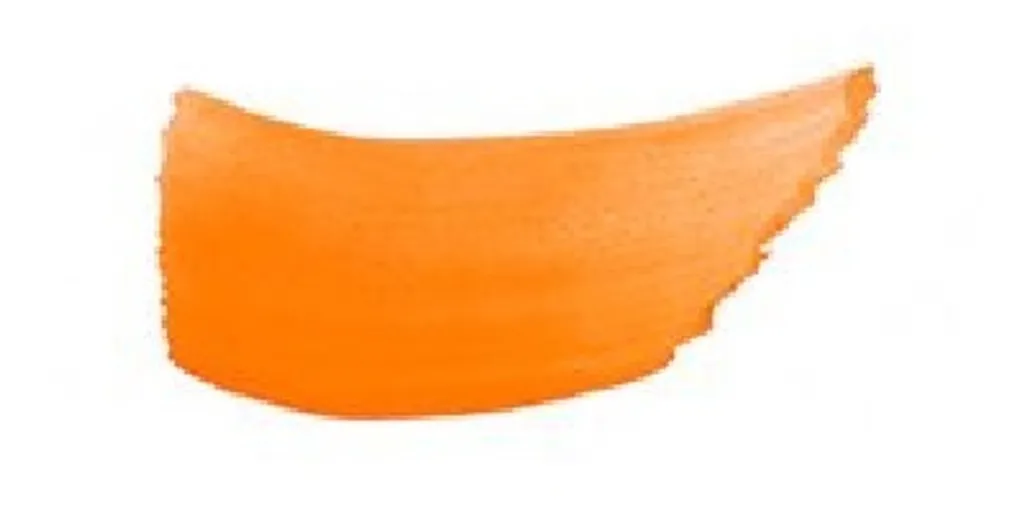The image features a vibrant, deep orange paint stroke splashed against a stark white background. The paint, reminiscent of the color of a rich orange peel or even a slightly more vibrant hue than macaroni and cheese, stretches from the left side to the right in a curved rectangular shape. The left edge forms a more solid rectangle, while the right edge appears ragged and unfinished, giving the impression of a spontaneous, unintentional brushstroke. The overall effect is somewhat abstract, lacking a discernible pattern or form, creating a simplistic yet striking visual contrast on the blank canvas.